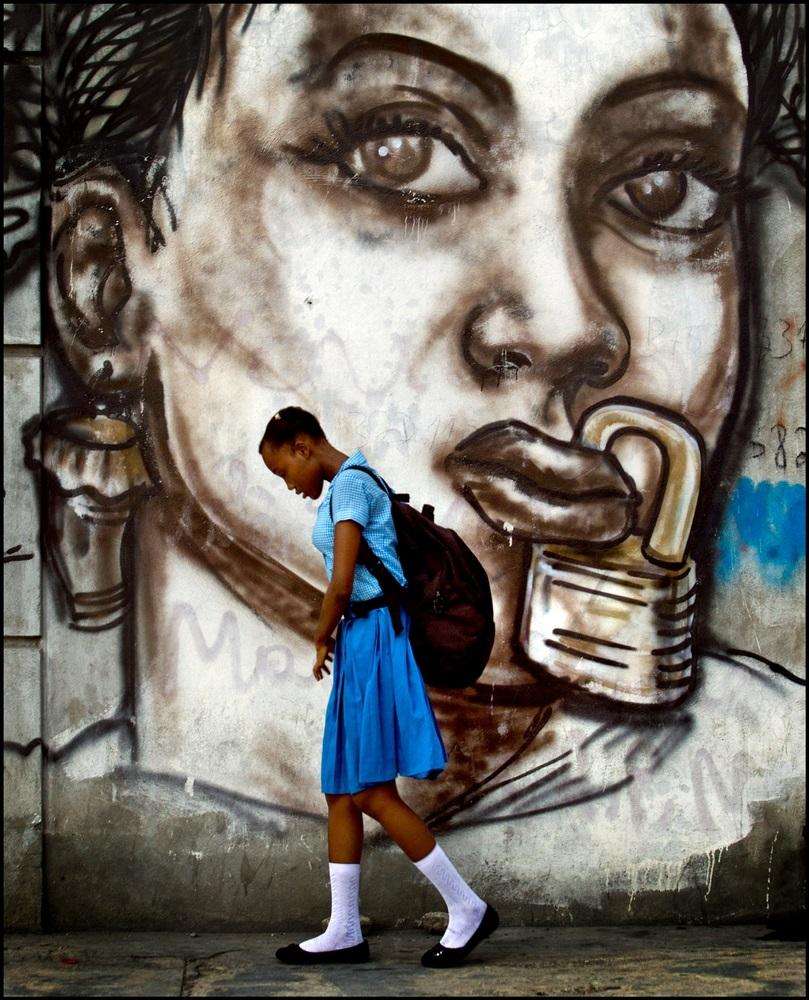In this evocative image, a young schoolgirl is walking from right to left in front of a mural that spans a gray concrete wall. She wears a slightly lighter blue collared shirt with short sleeves and a knee-length, darker blue pleated skirt, completing her outfit with tall white socks and black flat shoes. Her short, nearly shaved hair frames her downward-tilted head, giving her a somber appearance as she gazes at the ground. A very large maroon backpack, filled to capacity, is slung over her shoulders. The mural behind her features an African American woman with sorrowful, large eyes gazing intensely toward the viewer. The woman's stringy, short black hair falls over her left ear, adorned by a peculiar earring resembling a plastic-wrapped cup. Her protruding lips are pierced by a silver and brown padlock, symbolically sealing her mouth shut. This poignant artwork serves as a striking background to the girl's pensive walk along a dirty, broken sidewalk.